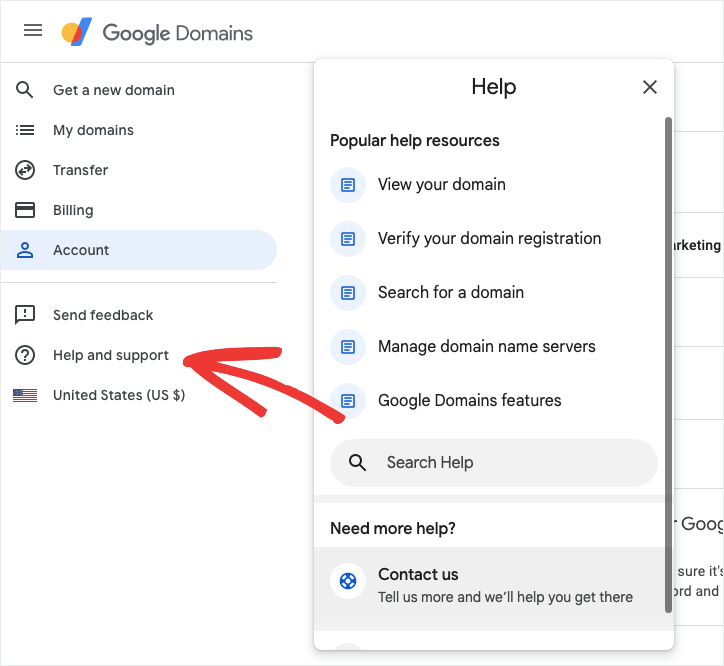Sure, here's a cleaned-up and more descriptive caption:

"In the upper left corner of the image, there is an orange and red circular logo with a blue line to the right, reading 'Google Domains.' The screenshot is divided into two sections. On the left side, there is an option to 'Get a new domain,' accompanied by a magnifying glass icon. Below this, the menu lists 'My domains,' 'Transfer,' 'Billings' (featuring an image of a credit card), 'Account,' 'Send feedback,' 'Help and support,' and 'United States US dollar,' which is represented by an illustration of a red, white, and blue flag. A red, edited arrow is pointing to the 'Help and support' option.

On the right side of the image, text is displayed vertically from top to bottom, listing 'Help,' 'Popular help resources,' 'View your domain,' 'Verify your domain registration,' 'Search for a domain,' 'Manage domain name servers,' and 'Google Domains features.' Below this list, there is a help box. Under the help box, it reads 'Need more help? Contact us,' followed by 'Tell us more and we'll help you get there.'"